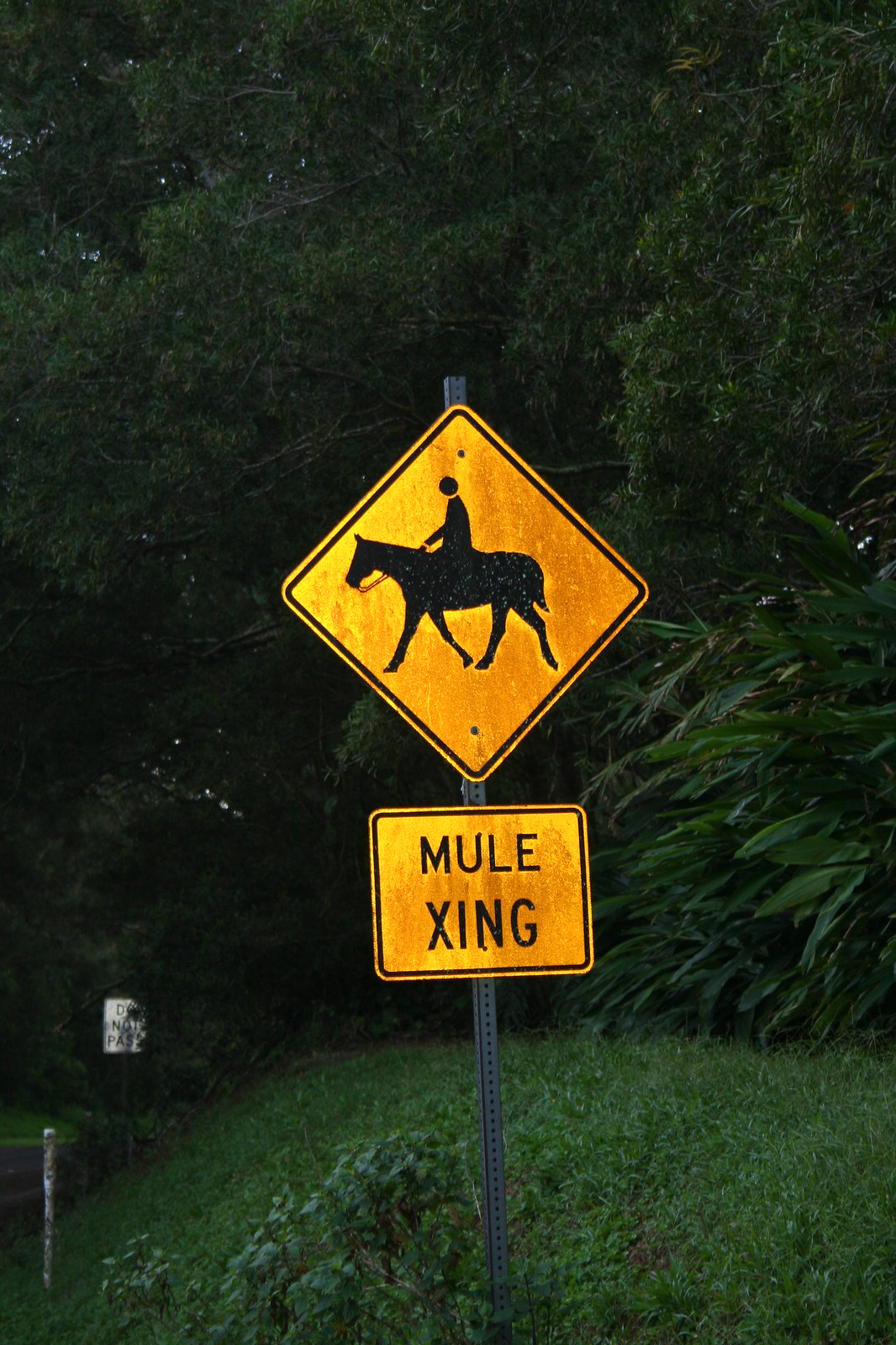This vibrant outdoor photograph, taken in portrait orientation, captures a scene set on a lush, green hilly surface teeming with vegetation. The background is dominated by dense, tall green trees intermingled with green bushes, which stretch all the way to the top of the image. Scattered around the base of the image, green grass and spiky plants further enrich the verdant landscape.

In the center of the photograph, a prominent yellow caution sign attached to a thin metal post draws immediate attention. The sign's diamond shape is affixed halfway up the post, presenting the black silhouette of a mule and rider. Below this, a rectangular yellow sign, slightly weathered with hints of rust, reads "Mule Crossing" with the abbreviated "X-I-N-G" clearly visible. Just beyond the primary sign, a small sterile bar protrudes from the ground, and something white can be observed in the distant background, adding to the intricate details of the scene.